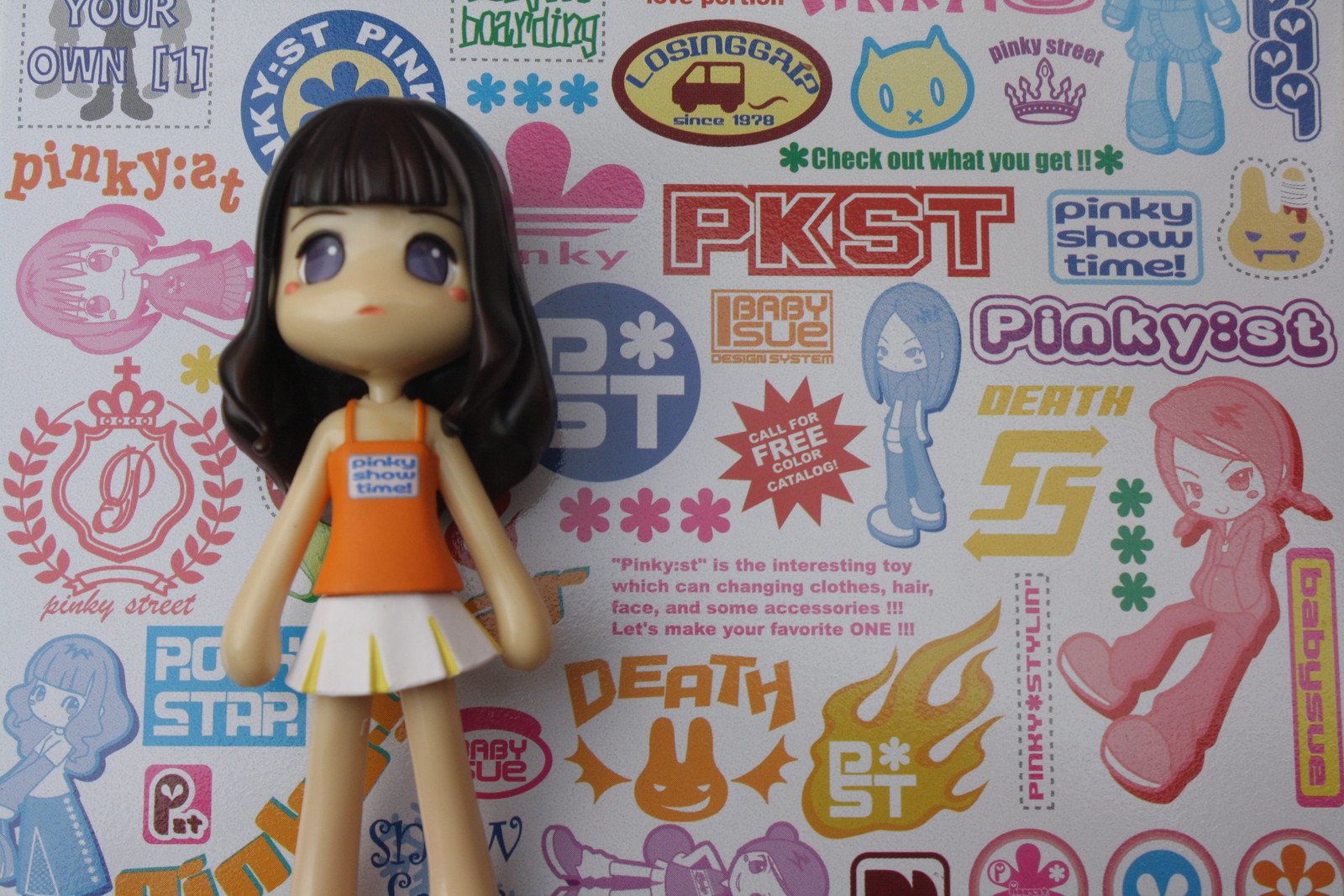The image depicts a central doll designed in a chibi anime style, characterized by a large, bobblehead-like appearance with expressive blue eyes and dark black hair that falls past her shoulders. She has a tan complexion and wears an orange tank top with the words "Show Time" partially visible. Her skirt is reminiscent of a cheerleader's outfit, predominantly white with yellow accents. The doll's arms and legs are articulated, although her hands lack detailed fingers, and her feet are not visible in the frame.

Surrounding the doll, the background is a vibrant collage of advertisements and promotional content for similar dolls and accessories. This backdrop features a multitude of colors, including pink, blue, orange, and red, and includes text such as "PKST," "Pinky Street," "Death," "ST," "Rock Star," and "Call for a free color catalog." The overall presentation appears as a photograph of a miniature doll with various other similar characters displayed behind her, promoting the customization options for these toys, which can change in color, hair, face, and accessories. The text and promotional materials suggest that the advertisements may not be authored by a native English speaker, adding an eclectic and somewhat whimsical element to the display.